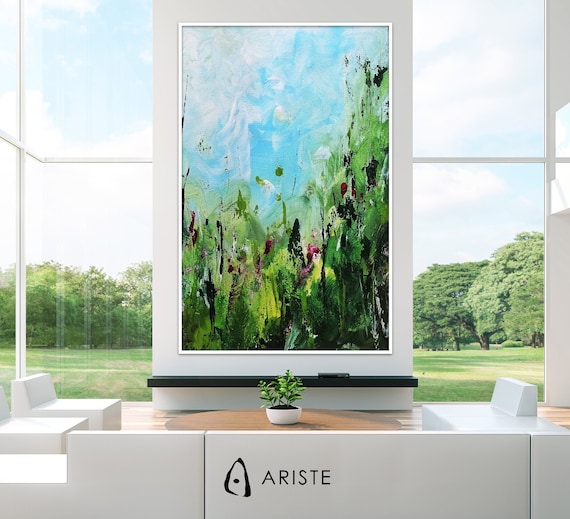The image is a highly detailed 3D rendering of a modern living room or office space, showcasing a sleek, contemporary aesthetic. At the center of the composition is a large framed painting, depicted with abstract green splotches that resemble tropical vegetation against a light blue sky. The painting stands against a wall made entirely of large white-framed glass panels, with views of a lush green lawn and various trees outside, under a partly cloudy sky with hints of blue. The floor is a rich wood finish, and the furniture consists of blocky, geometric armchairs and couches made of a plastic-like material. A round coffee table with a small potted plant sits in the middle of the room. In the bottom left corner of the image, the logo "ARISTE" is prominently featured, possibly attributing the artwork or design to a particular creator or company.